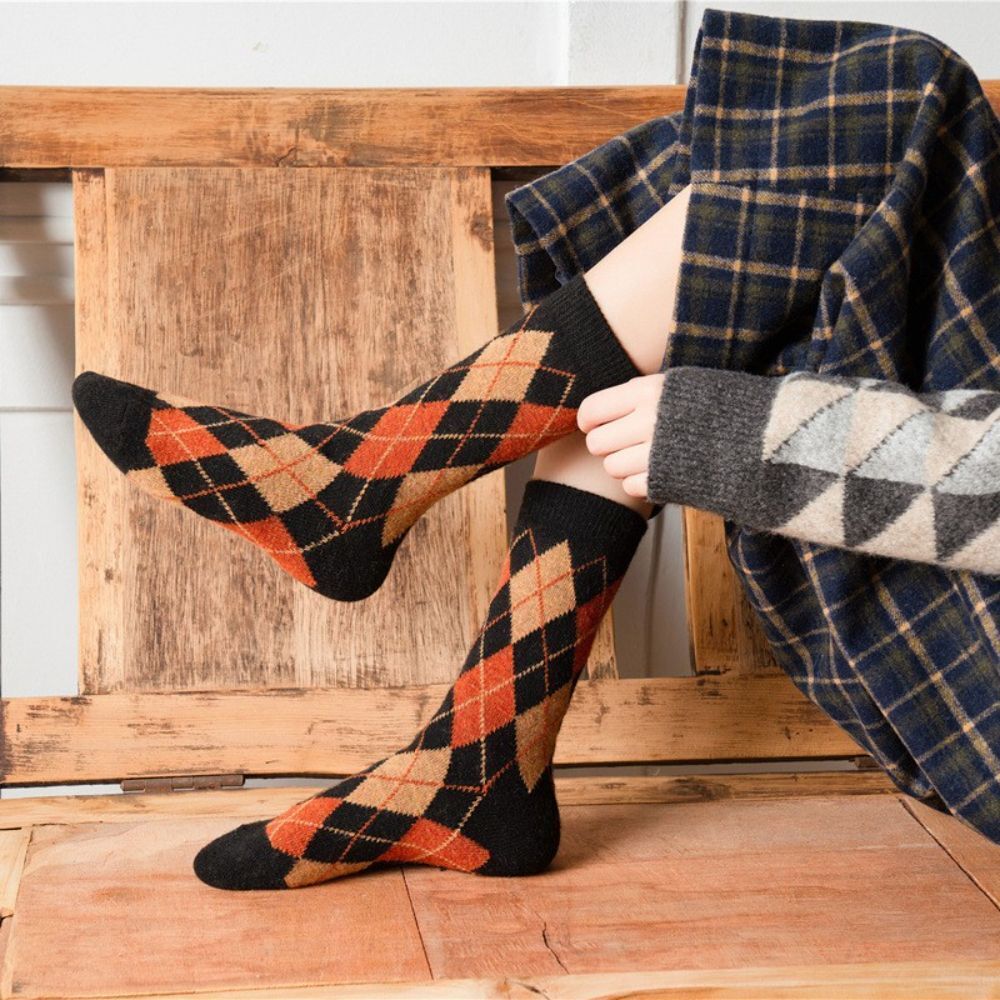The image shows a woman from the waist down, captured from the right side, with her lower legs extending to the center of the frame. She is seated on a brown wooden floor in front of a white wall, with a brown wooden bench or shelf in the background. She is wearing cropped white pants adorned with dark blue and light brown square patterns. Her grey sweater features a square-shaped design in white, light blue, and grey. The woman is putting on a pair of argyle socks that are black with diamond shapes in yellow, orange, and possibly light brown. One foot is raised with the sock partially on, while the other foot, fully socked, rests on the wooden bench. The overall scene exudes a cozy, autumnal feel with the warm wooden tones and fall-themed socks against the neutral background.